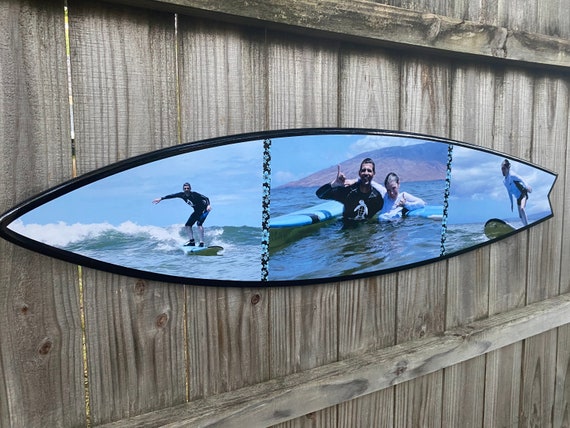The image showcases a weathered, grayish wooden fence, characterized by vertical planks reinforced with two horizontal support bars. Mounted on this aged fence is a rimmed black surfboard divided into three sections, each featuring its own photographic scene. The left quadrant portrays a man in a wetsuit surfing a wave under a vivid blue sky, his hands outstretched as he rides toward the viewer. The middle section depicts a man and a woman waist-deep in water, with a blue surfboard positioned nearby; the man in a black wetsuit gestures with a finger raised, while the woman in a white top looks downward. Adding a touch of detailed artistry, the separations between the photos feature a band with blue tropical flowers. The rightmost section of the surfboard presents a serene blue sky filled with clouds, the ocean, and a young girl in a white wetsuit and bikini bottom balancing herself with her outstretched arms. The overall color scheme blends natural gray tones of the fence with the blacks, whites, and blues of the surfboard and its photographic images.